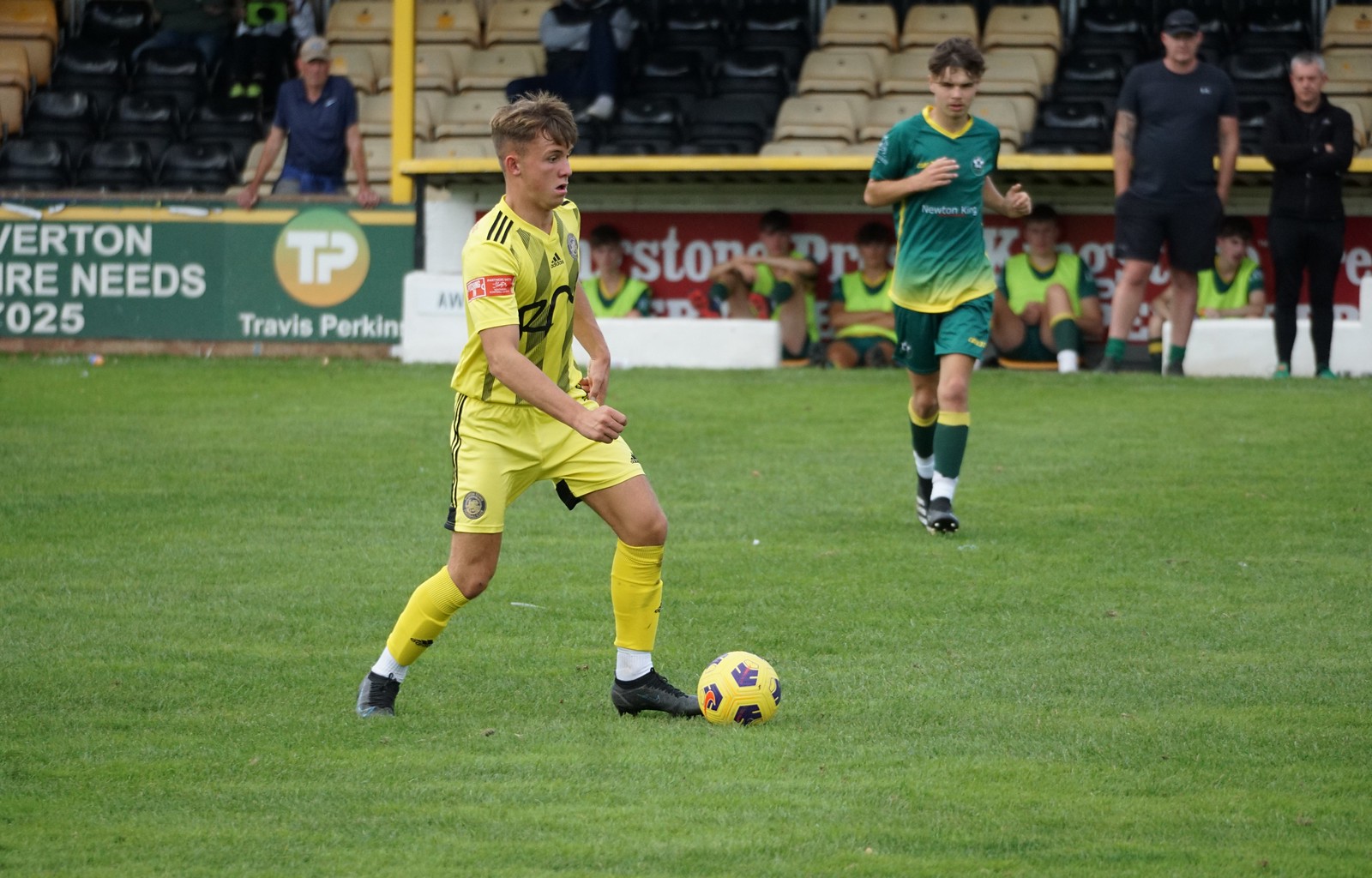In this detailed photograph of an English football game taken inside a sparsely populated stadium, the focus is on two players in the midst of action on the green grass field. In the center, a white male player with short blonde hair, shaved on the sides and long bangs at the front, is captured mid-kick of a yellow and black soccer ball. He is fully dressed in an Adidas neon yellow uniform, comprising a jersey with three black stripes on the shoulders, yellow shorts with three black stripes down the sides, yellow socks, black cleats, and a red captain's band on his right arm. Approaching him is another white male player with shaggy brown hair, outfitted in a green uniform with yellow trim on the shirt and socks, and green shorts. The stands in the background reveal black and tan seats with scant attendance—only one visible spectator dressed in blue standing amidst the empty rows. Close to the field, several players in green uniforms with bright green bibs and two coaches are seen in the bench area, which is slightly lower than the playing field.